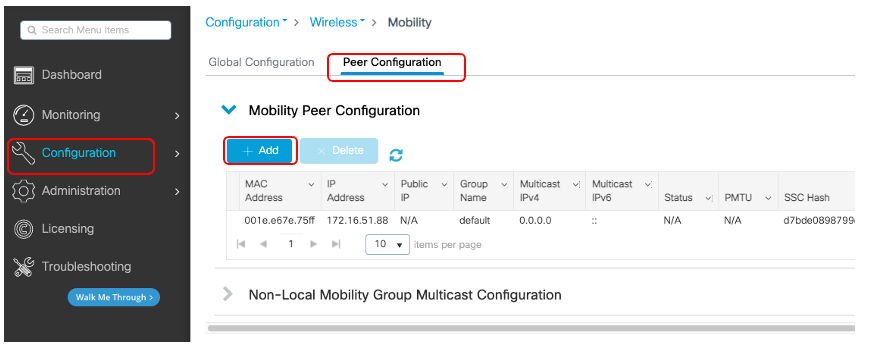**Detailed Caption:**

This image displays a web interface related to wireless mobility and configuration. At the bottom, bold black text reads "Non-local Mobility Group Multicast Configuration." 

In the upper left corner, a black sidebar contains several drop-down menus and a search bar allowing users to enter their information. The sidebar also provides navigation options labeled in white text, including "Dashboard," "Monitoring," "Configuration," "Administration," "Licensing," and "Troubleshooting." Additionally, there is a long blue button labeled "Walk Me Through."

At the top of the main section of the page, two tabs, "Configuration" and "Wireless," are highlighted in blue. Next to them, "Mobility" is marked in black. Below, sub-sections "Global Configuration" and "Peer Configuration" are listed with "Peer Configuration" outlined in red and featuring a blue underline. This indicates that the user has selected the "Peer Configuration" section.

Within the "Mobility Peer Configuration" area, the user interface displays options to add or delete configurations, both denoted in blue text. The "Add" button is highlighted with an orange outline. The section below lists fields for "MAC Address," "IP Address," "Public IP," "Group Name," "Multicast IPv4," "Multicast IPv6," "Status," "PMTU," and "SSC Hash." 

At the bottom of this section, pagination options are available, and the user has highlighted the "10," indicating they are viewing the last page of entries.

The user appears to be in the process of locating specific information within this peer configuration setup.